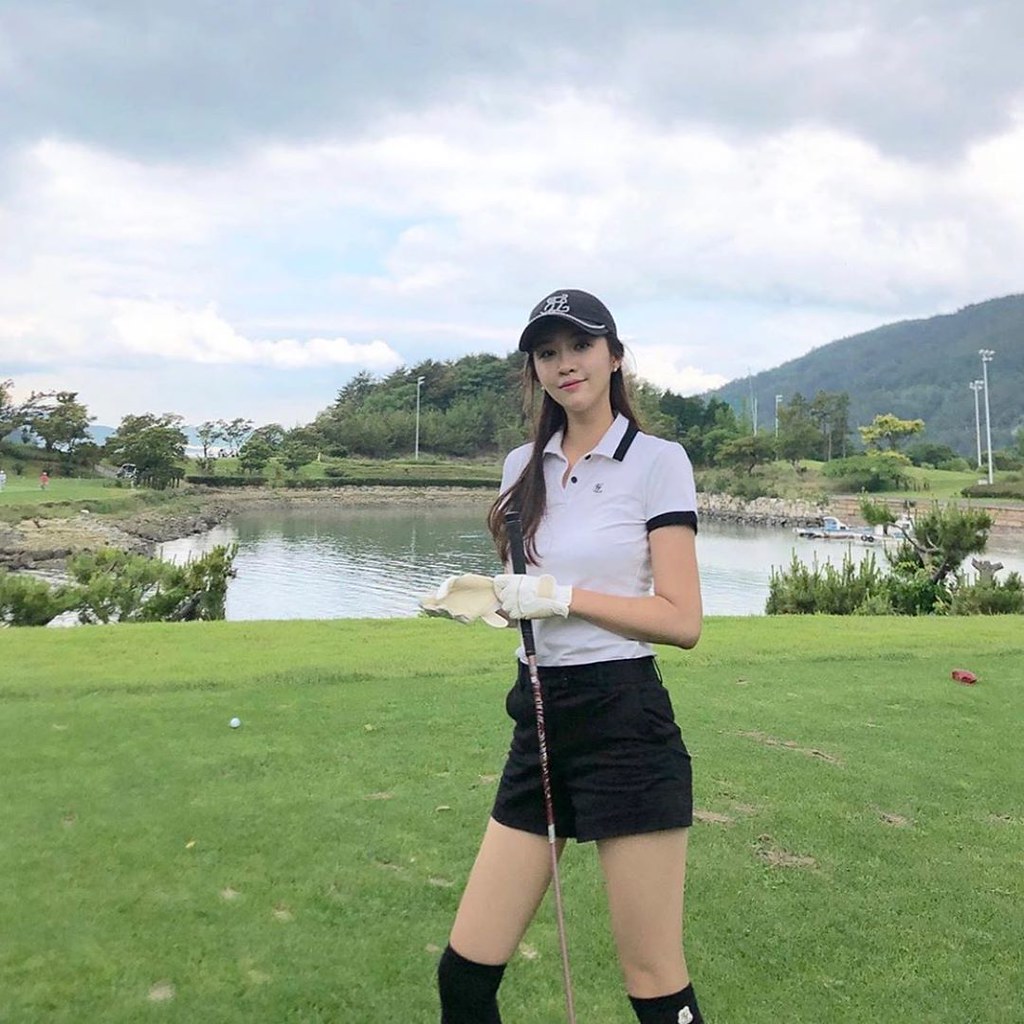This vibrant daytime photograph is a square-shaped, 6x6 inch snapshot taken outdoors, featuring an Asian girl centered and facing the camera on a golf course. Dressed in traditional golfing attire, she sports a black baseball cap with white lettering, a short-sleeved white polo shirt accented with black trim around the collar and cuffs, black shorts, and black knee-high socks. Her white golf gloves grip the handle of a golf club, suggesting an active moment on the course. The meticulously manicured green grass occupies the lower half of the picture, with a small white golf ball visible to her left at waist height. The background reveals a sprawling pond flanked by steps leading down to some boats on the right side, beyond which lie lush trees and mountains. A mix of blue sky and white clouds can be seen, with darker, rain-threatening gray clouds at the very top, adding a dramatic touch to the scene.